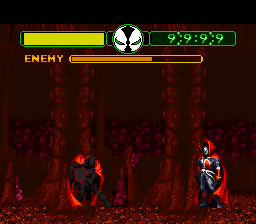The image depicts a screenshot from an early 2000s handheld video game, likely featuring characters from Spawn Comics. The overall background is a dark burgundy, interspersed with lighter brown elements that resemble posts, giving the impression of a grandstand filled with indistinct figures. At the top, there's a prominently displayed interface with a series of status bars and numerical indicators: a full yellow bar labeled "Enemy," a partially filled orange-yellow bar, and a black box highlighting the time as "9999" in bright green digits, all outlined with neon green accents. Dominating the scene are two Spawn-like characters. 

The character on the left wears an all-black outfit with a striking neon red cape and shield, adorned with a matching red trim. This figure stands in a darkened forest-like setting with tree trunks and reddish-brown soil. The protagonist, positioned on the right, dons a predominantly black suit accentuated with red designs on the chest and gloves, and a mask matching the one shown between the status bars above. This character is also enveloped in a vivid red cape with high collars extending past their head, adding to the dramatic atmosphere of this tense confrontation.